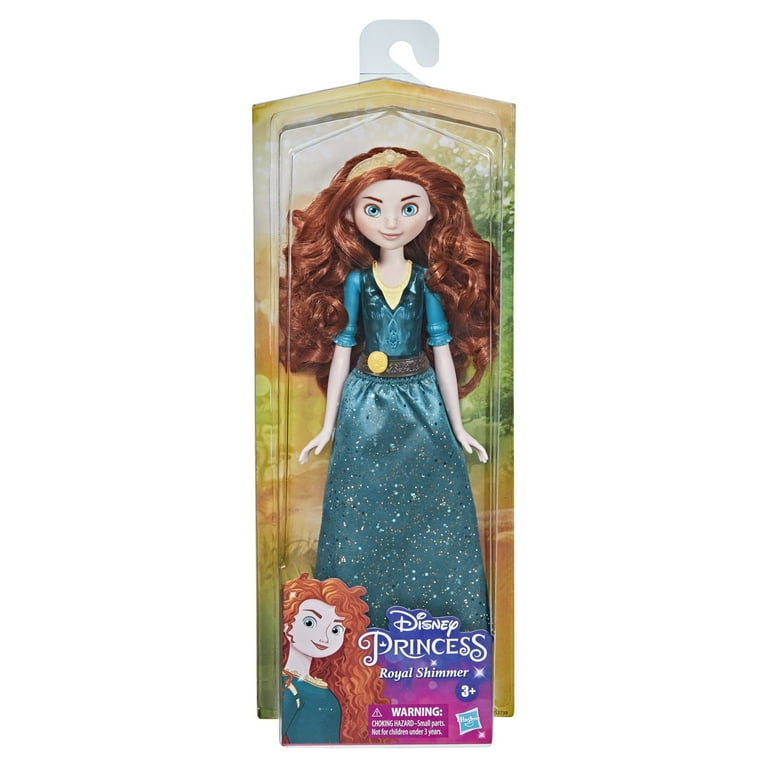This photograph captures a Disney Princess Royal Shimmer action figure designed for children aged 3 and up, encased in its original plastic packaging. The packaging features the Disney logo in purple and pink at the bottom, along with a choking hazard warning. The doll is a beautifully detailed representation of a princess with long, bright red hair that cascades around her shoulders and a gold crown adorning her head. She has striking green eyes and rose-colored lips, radiating elegance. The princess is dressed in a sparkly turquoise blue dress that flows gracefully to her feet, embellished with shimmering sprinkles of blue, green, and turquoise hues. Underneath the dress, she wears a yellow shirt, and a black belt with a prominent gold circle accentuates her waist. Additionally, she sports a gold necklace, complementing her regal appearance. The box also includes an image of the princess and features a hook at the top, indicating it was designed to be displayed hanging in stores.